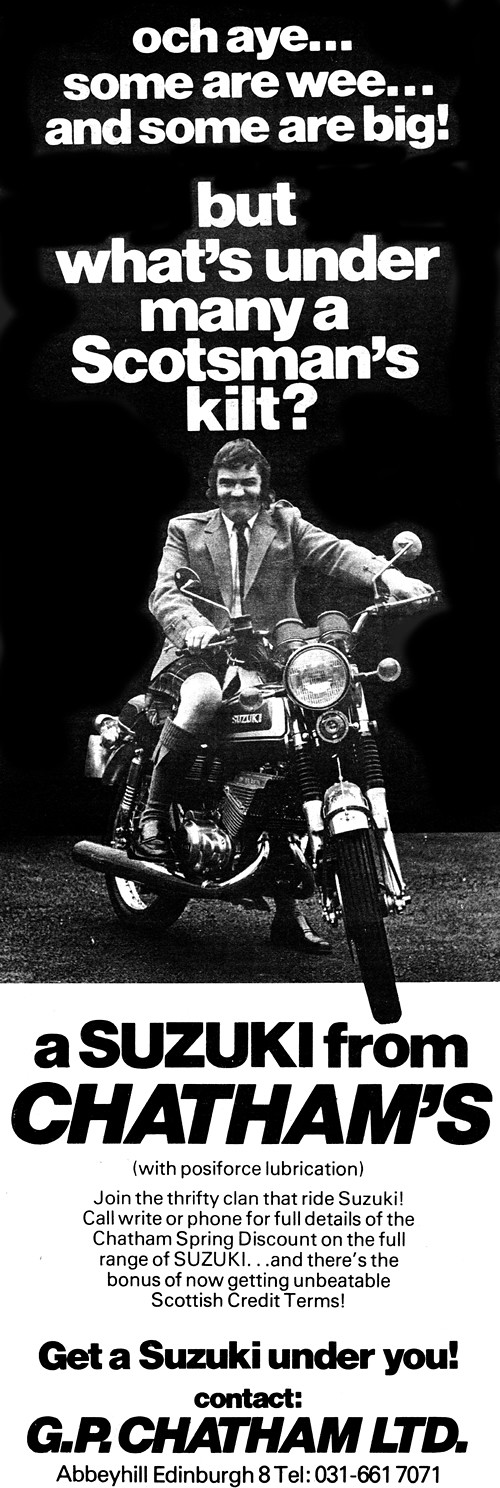This black and white advertisement for Suzuki Motorcycles features a striking image of a Scotsman sitting on a Suzuki motorcycle against a black background. The Scotsman is dressed in a traditional kilt, complemented by a light suit, a dark tie, and tall black boots. His hands are confidently placed on the handlebars, and the front wheel of the motorcycle is turned to the left, adding a dynamic feel to the pose. 

Bold white text at the top reads, "Oach aye, some are we and some are big, but what's under many a Scotsman's kilt?" In bold text beneath the image, it proudly states, "A Suzuki from Chatham's." Followed by a smaller caption urging, "Join the thrifty clan that rides Suzuki. Call or phone for full details of the Chatham Spring Discount on the full range of Suzuki." Additionally, it highlights the "unbeatable Scottish credit terms," ensuring an enticing offer. The advertisement concludes with a call to action, "Get a Suzuki under you! Contact GP Chatham Limited in Aberdeen and Edinburgh," indicating locations and contact information for potential buyers.